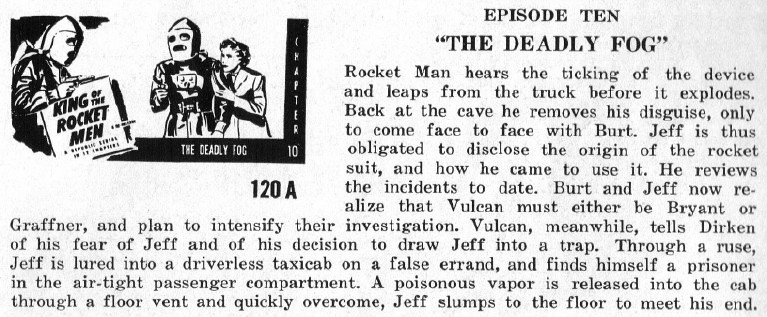This black-and-white newspaper clipping appears to be an old serialized comic or story extract, specifically Episode 10 titled "The Deadly Fog." The layout features a picture on the left of Rocketman standing with a woman, captioned "King of the Rocketmen." The narrative tells of a perilous episode where Rocketman, known as Jeff, hears the ticking of a device and leaps from a truck just before it explodes. Reaching safety at a cave, he removes his disguise and encounters Bert, compelling him to disclose the origin of his rocket suit.

Jeff reviews past incidents, leading him and Bert to suspect Vulcan is either Bryant or Gaffner, prompting them to intensify their investigation. Meanwhile, Vulcan, fearing Jeff, plots to trap him. Jeff is tricked into entering a driverless taxi and becomes trapped in the airtight passenger compartment. Poisonous vapor is released through a floor vent, and Jeff, quickly overcome, slumps to the floor, seemingly meeting his end.